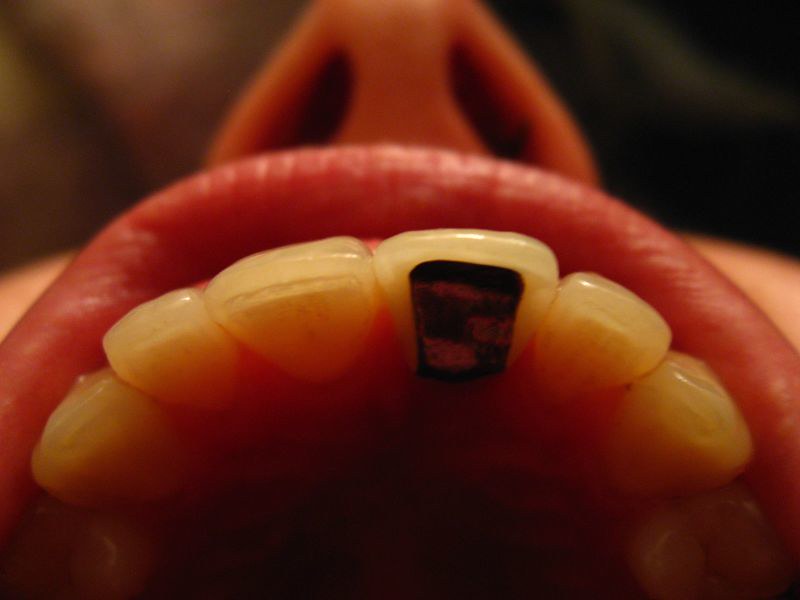This is a close-up color photograph of a person’s open mouth, captured in landscape orientation. The image prominently features the upper row of the person's teeth and the upper lip towards the bottom. Underneath one of their front teeth, a silver rectangular object, which appears to be some sort of implant or decal, is visible. The viewer can also see the individual's nostrils at the top of the image. The backdrop and areas behind the lips and teeth are blurred and hazy, likely to keep the focus on the main subject. The photograph is characterized by its realism and representational style, showcasing intricate details of the teeth and mouth.